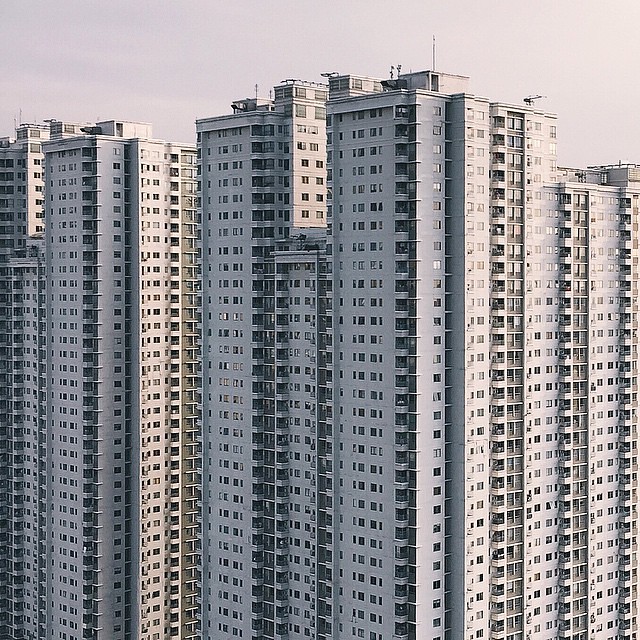The image features several extremely tall, white, high-rise buildings that dominate approximately 95% of the frame. These rectangular-shaped buildings are arranged closely together, creating a somewhat cube-shaped configuration. The structures have a uniform, symmetrical appearance with over 30 to possibly 50 floors, and their facades are covered with numerous small, black square windows. The buildings seem somewhat bland and are rendered in a grayish-white color, with shadowed portions appearing slightly blue. At the top, some buildings have small notches and antennas, adding minor variations to their otherwise monotonous design. The upper 5% of the image captures a grayish-white sky with patches of clouds, through which sunlight permeates, particularly illuminating the right-hand side of the buildings while leaving other sections in shadow. The overall scene conveys a sense of towering urban uniformity against a muted sky.